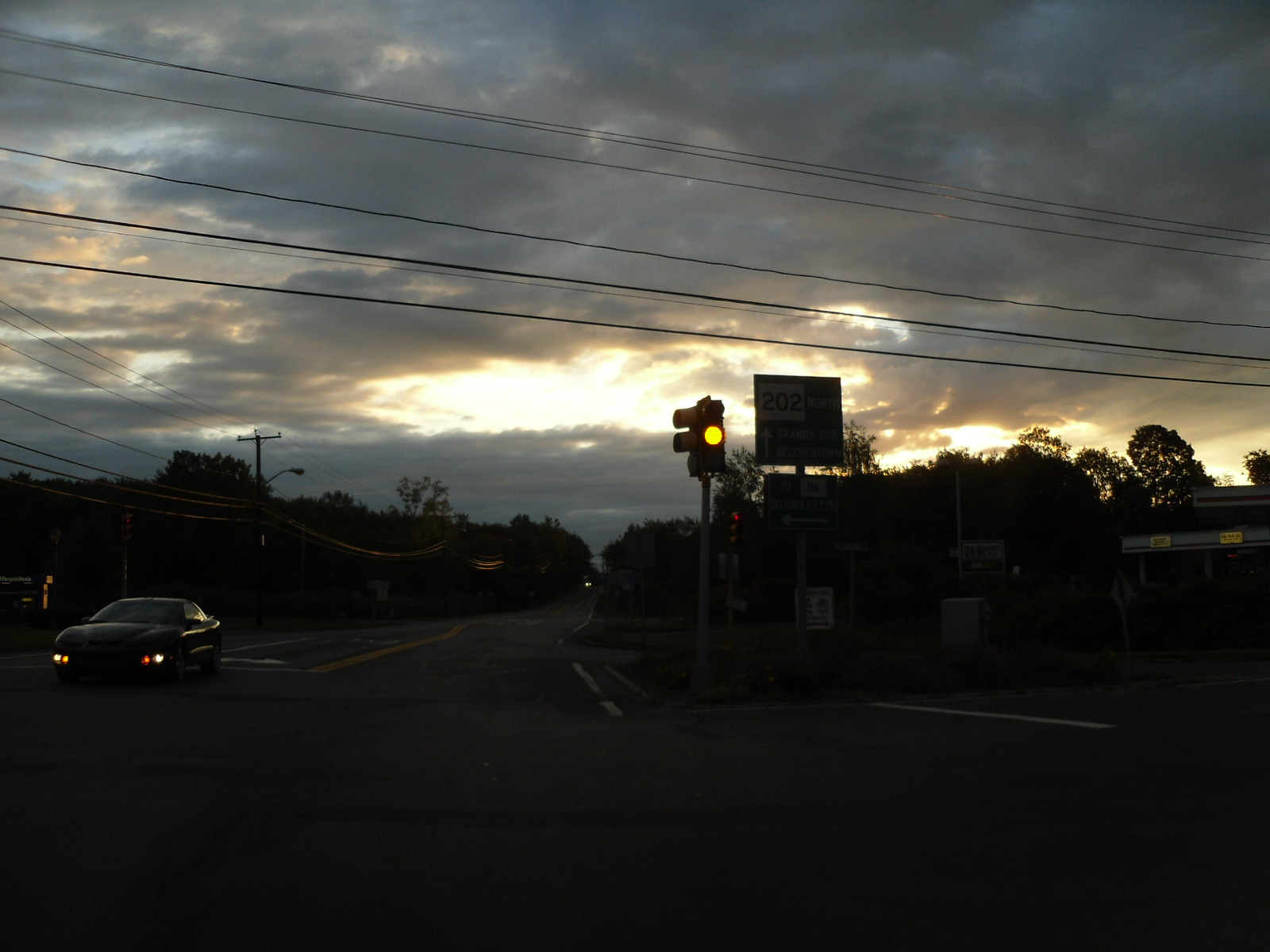The image captures a dimly lit landscape scene at an intersection, emphasizing the dramatic interplay of light and shadow. On the left side of the image, a black sports car approaches a stop sign, its yellow and orange headlights glowing under an overcast sky. The car sits at a junction marked by a solid yellow line, leading the viewer's eye down a long street flanked by dark, green forestry. Amidst the moody ambiance, a brief sliver of white-yellow sunlight peeks through the cloudy sky, casting a faint glow over the scene.

Dominating the center is a yellow streetlight and a road sign mounted on a grey pole, bearing dual arrows with the top one pointing upward and the bottom one to the left. Though the text on the signs is blurry, the details evoke a sense of navigation and direction. To the right of the image, a gas station with white poles and decals adds a splash of industrial calm against the natural backdrop.

The scene is further textured by electrical power lines that stretch horizontally across the image and crisscross down the side roads, contributing to the urban feel. The street layout is complemented by a mix of yellow and white road markings, and the entire image has a dark, almost melancholic tone, either due to camera settings or the overcast conditions. The melancholic tone is capped off by a traffic light showing amber, indicating the fleeting moments of dusk. In the distant background, faint headlights hint at another vehicle approaching, adding depth and a sense of continuity to the otherwise serene and static setting.